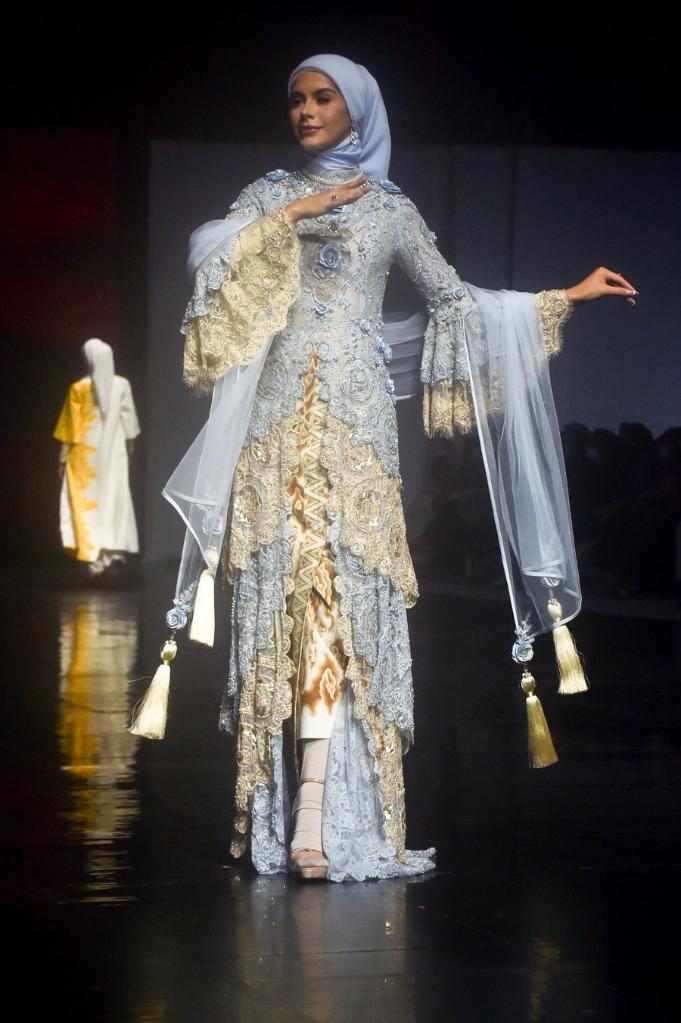In this color photograph, the setting appears to be an indoor fashion show with a black stage floor. In the foreground, a captivating woman with possibly Middle Eastern features walks confidently towards the photographer, her face adorned with subtle makeup and a closed-lip smile. She's dressed in an intricate, floor-length flowing blue dress that showcases elaborate details such as large, lacy sleeves, sheer fabric, and dangling tassels. Her outfit is interspersed with hints of off-white and golden accents. Complementing her dress, she wears a light blue headdress and scarf, styled like a hijab, which adds a touch of elegance. Her brownish shoes peek out from beneath the layers of her gown, and a ring sparkles on her hand, adding to her sophisticated appearance.

In the background, another model walks in the opposite direction, fading into the dark stage. This secondary figure is clad in a long, flowing white dress subtly accented with yellow and complete with a matching white headscarf. The black backdrop adds contrast, making the white of her dress and headscarf, as well as her shadow, stand out starkly, enriching the image's visual depth. The overall atmosphere exudes a sense of refined style and elegance, characteristic of a high-end fashion show.